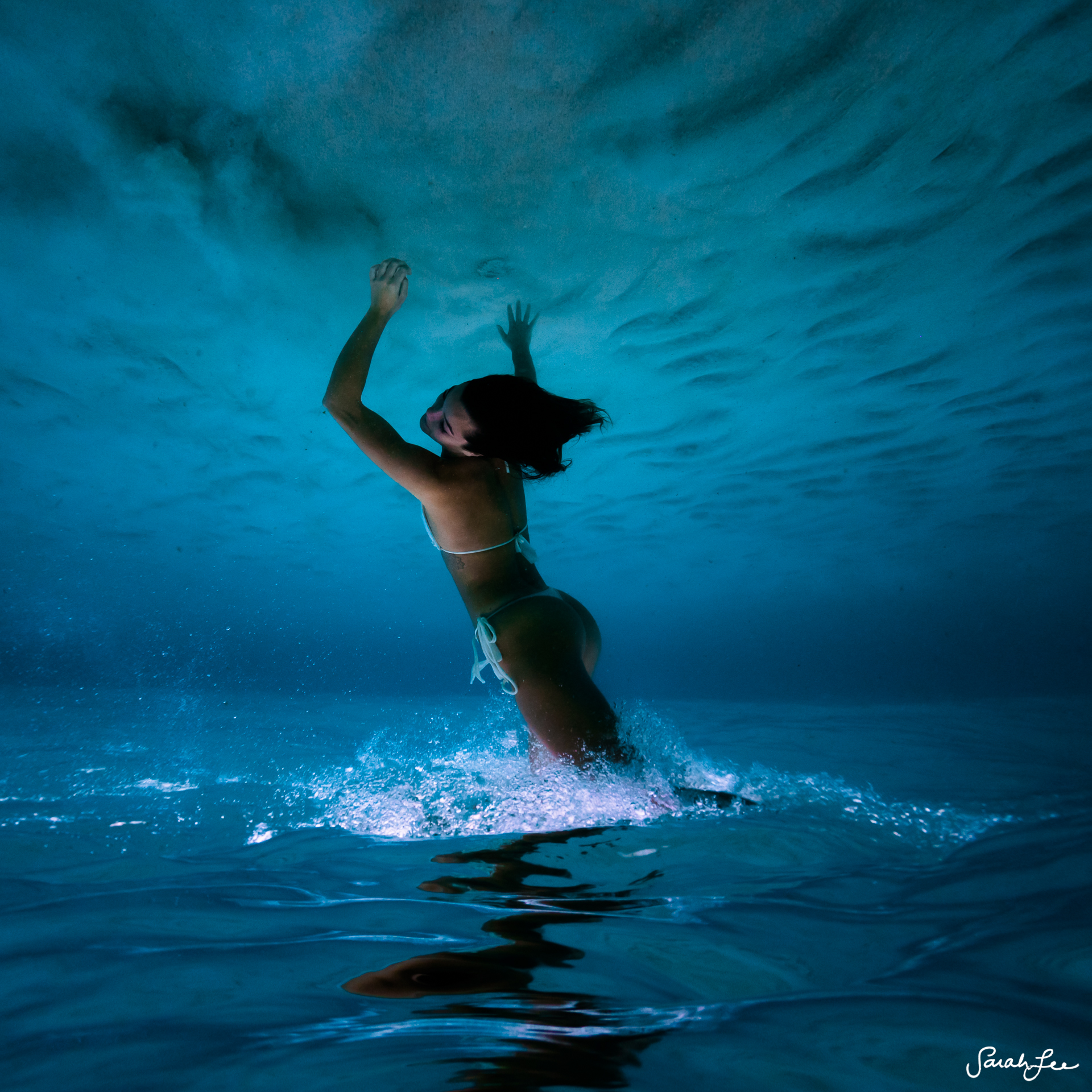The image depicts a woman in a white string bikini with dark hair, appearing to leap out of dark, shadowy water, her arms stretched upward as if reaching for the sky. The scene is surreal, with an upside-down perspective that makes it seem like she is both diving and emerging from the water simultaneously. Her hair flows dynamically in the water, and splashes around her thighs indicate the point where she broke the water's surface tension. The background features very dark blue and green clouds, which add to the image's moody and somewhat eerie atmosphere. The photo is dimly lit with low contrast, creating a heavy, dark ambiance, punctuated only by the splash of water around her. At the bottom right corner, the image is signed by the artist, Sarah Lee.